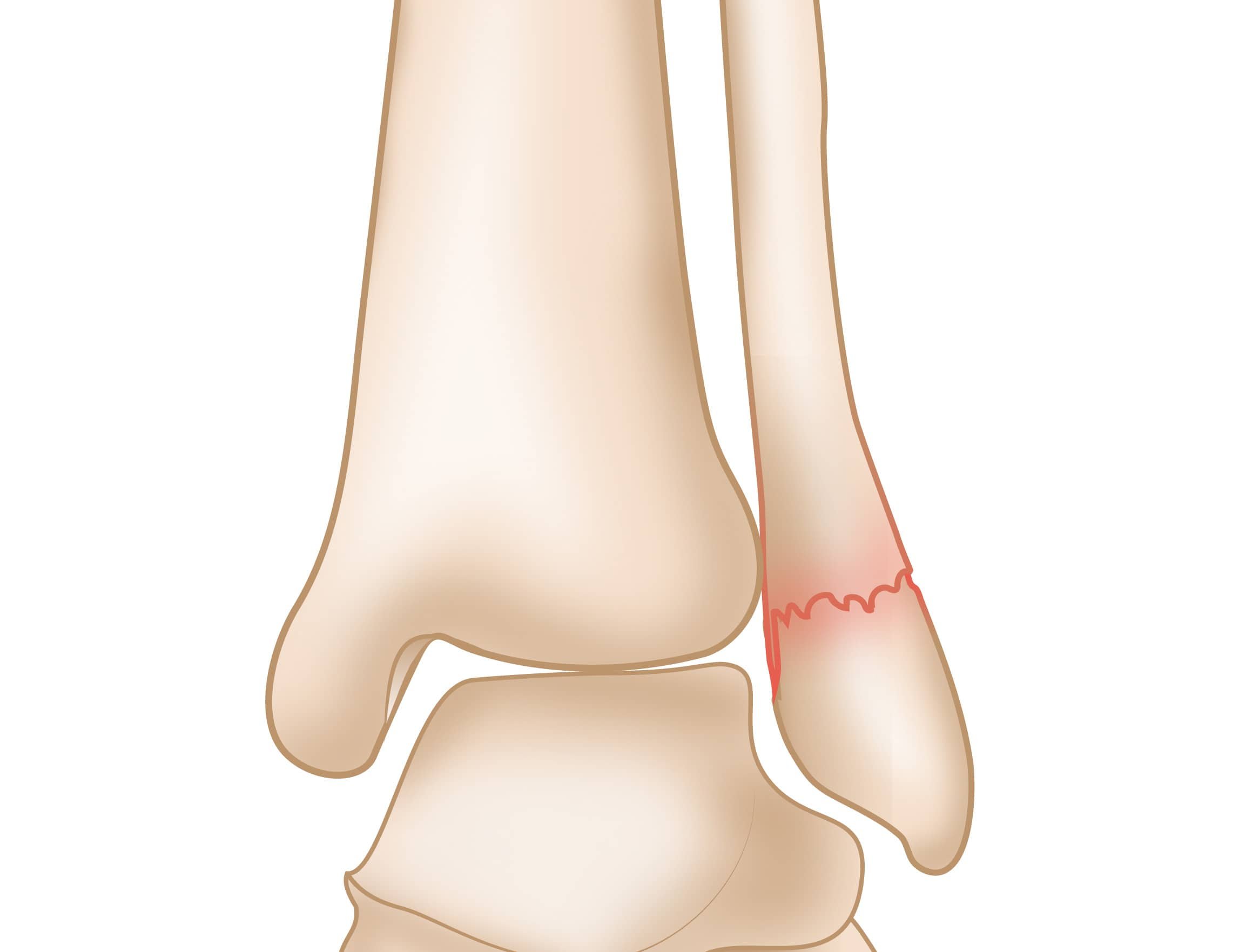This detailed illustration presents an elongated, unbordered depiction of three interconnected bone sections, set against a stark white background. The bones, which are possibly human but not definitively identified, exhibit a natural white hue with tan edges. The top section is broad, the middle section is notably thin and long, and the bottom section is wide but partially cut off, hinting at a larger structure outside the frame. A prominent red zigzag line indicates a fracture in the lower wide bone, surrounded by redness emphasizing the break. Despite the lack of explanatory captions or labels, the image clearly focuses on detailing the fracture and the connection points among the bone sections.